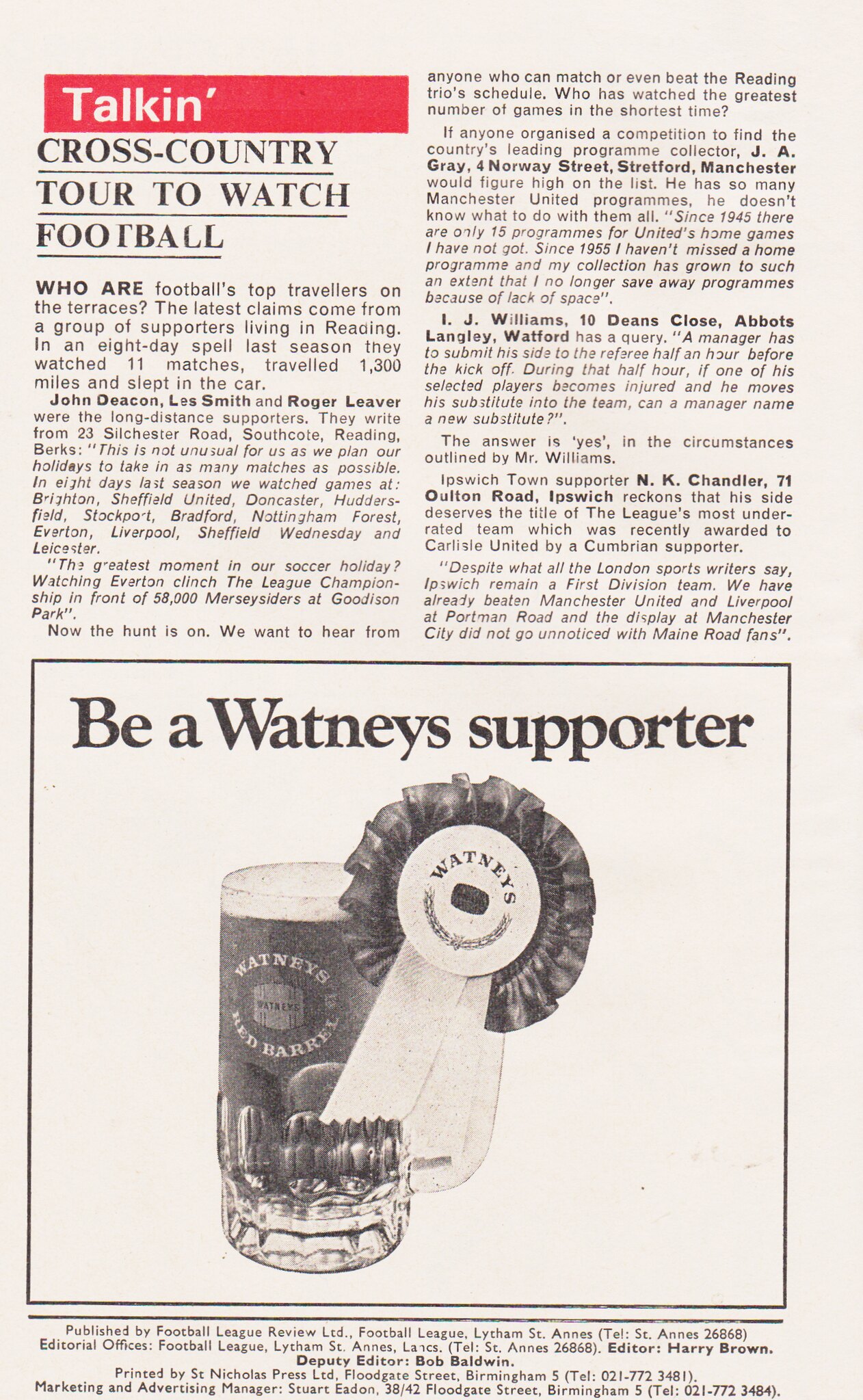The image depicts an old newspaper or magazine article on an off-white, almost gray-beige, worn-out page. In the upper left corner, there's a red stripe with the word "TALKIN" in bold white letters. Beneath this stripe, the headline in black text reads, "Cross-country tour to watch football." The upper half of the page contains a two-column article, with black text continuing down the first and second columns. Below the article, there is a large black-and-white photograph framed by a thin black border. The top of the photograph includes a prominent caption: "Be a Watney supporter." The photograph itself shows a tall glass of beer labeled "Watneys Red Herald" beside a decorative fabric ribbon that says "Watneys," possibly in blue or black. The ribbon appears ruffled around the edges and extends down in a fabric strip. At the very bottom of the page, there's a line of very small black text that is difficult to read due to its fine print.